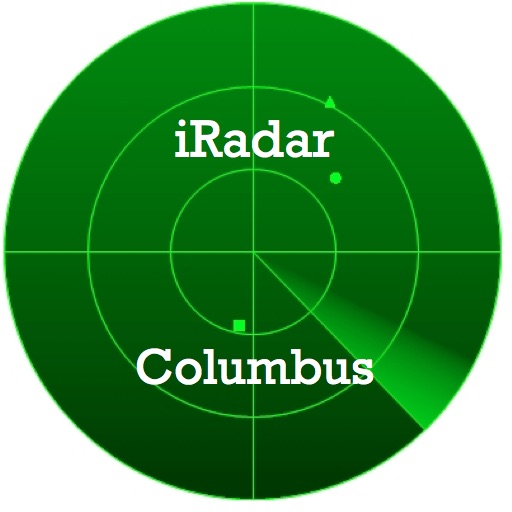The image depicts a radar illustration dominated by a large, brilliant green circle with intricate details. The circle features a vertical line and a horizontal line intersecting at its center, creating a cross that dissects the circle into four equal sections. Within the main circle, two smaller, concentric circles are highlighted in lighter green, contrasting against the darker green background. Various objects detected by the radar are represented by a light green square, dot, and triangle. A scanning line, reminiscent of a watch hand, sweeps around the circle, indicating active scanning areas. The words "IRADAR" in white letters are prominently displayed at the top center of the main circle, with "Columbus" similarly positioned below, also in white. This detailed radar illustration combines various shades of green and precise geometrical elements to convey a sophisticated tracking mechanism.